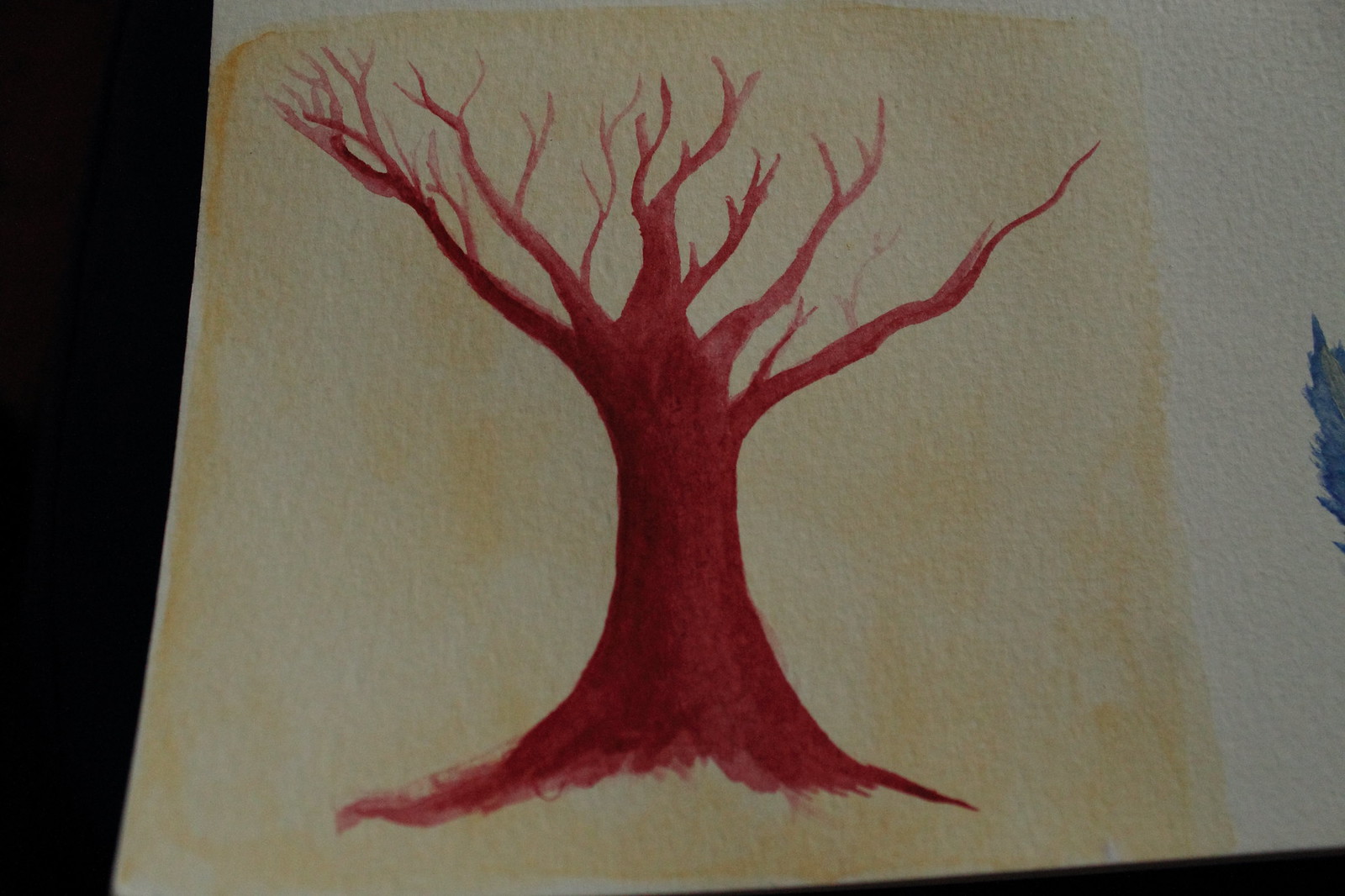This descriptive caption for the watercolor painting synthesizes the shared and detailed information from the different perspectives:

"This artwork is a watercolor painting created on a thick, textured white paper. The left side of the paper features a very light wash of brown, creating a soft background that transitions into a beige color towards the center. Dominating the scene is a solitary tree situated in the middle of the page, depicted with intricate detail. The tree is brown, devoid of leaves, showcasing a sturdy trunk with six large branches that extend into numerous smaller twigs, giving it a complex silhouette. The tree appears to almost float, as there is no grass or ground depicted beneath it. Off to the right, the edge of the paper is white, and just peeking in from this side is a section with green and possibly purplish squiggles, hinting at the presence of another tree or some abstract design. The paper itself lies against a dark black background, highlighting its textured surface and the delicately painted tree."